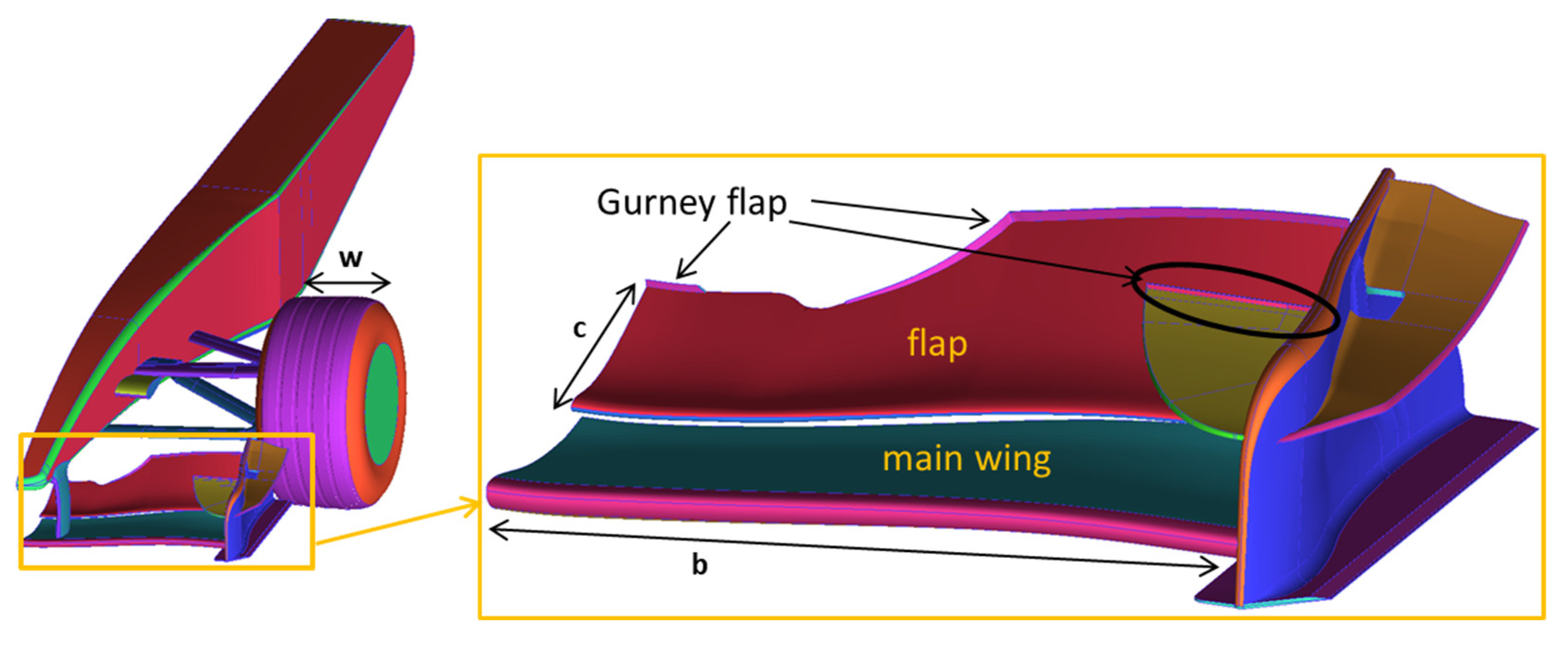This detailed informational diagram appears to depict the elements and assembly of a Gurney flap, likely used in aerodynamic contexts, such as on an airplane. The diagram features various components identified with distinct colors: green, red, purple, orange, and blue. Central to the diagram is a wheel, connected to a plank that may indicate part of a wing structure, and a close-up depiction of the Gurney flap labeled in different sections. The Gurney flap is annotated with labels and color-coded parts, including a red flap and a dark blue, or nearly black, portion marked as the "MAIN WING," trimmed in bright dark pink. On the right side, the diagram outlines several locations where the Gurney flap is connected to the main wing, demonstrating how it is affixed structurally. Additional components, such as a blue side piece and a brown protruding piece, are also highlighted. Arrows and labels like "C" and "D" point to specific areas, providing further clarification. A smaller inset diagram on the far left illustrates a close-up of the wing with a purple tire, encircled in orange and a green center, integrating these components into the larger structure, and indicating their relative positions and connections within the overall assembly of the Gurney flap and main wing.